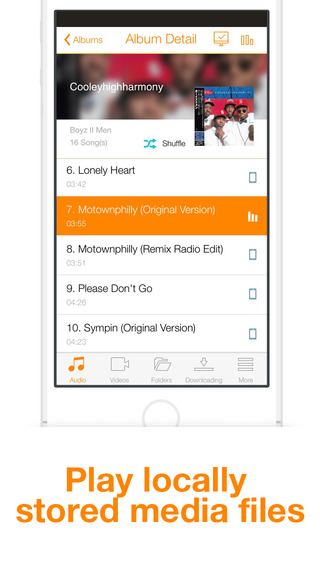The image displays a cellphone screen predominantly in a sleek, modern design, with a notable lack of physical buttons on the sides. A standout feature is the round button situated at the bottom left corner of the device. The screen is showcasing a music player interface, specifically an album overview for "Cooley High Harmony" by Boyz II Men. 

In the album's tracklist, notable songs include "Lonely Heart" listed as track seven and "Motownphilly (Original Version)" as track eight, followed by "Motownphilly (Remix Radio Edition)" at track nine, and "Please Don't Go" at track ten. Additional media options like audio, video folders, and downloading features are visible. 

Below these options, on a clean white background with orange text, there's a prompt that says, "Play locally stored media files." The interface predominantly features colors such as orange, black, gray, and white. The album art for "Cooley High Harmony" incorporates vibrant reds and blacks, while another visible CD cover blends red and blue hues. There are touches of green within the interface, including a green shuffle button icon. 

Overall, the display is a dynamic mix of functionality and aesthetics, emphasizing ease of use and visual appeal.